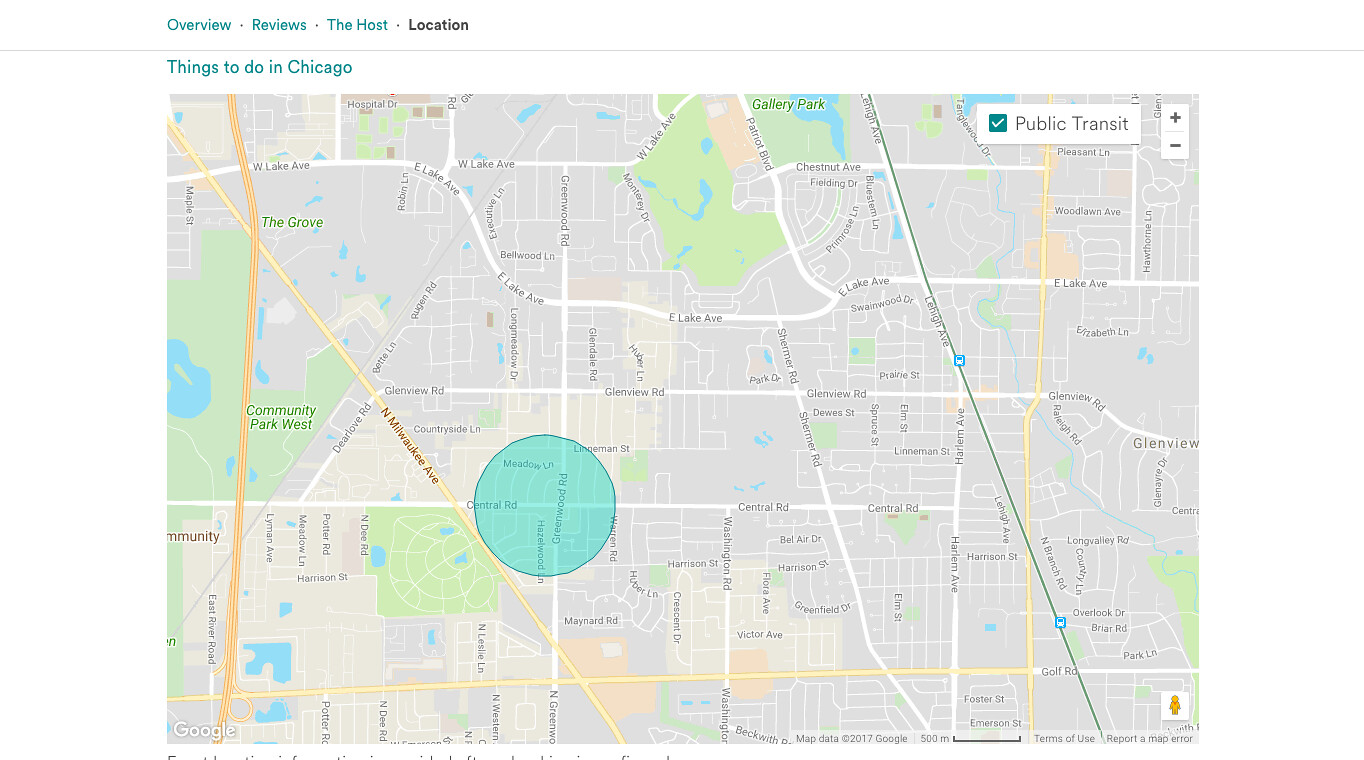This image is a detailed screenshot from Google Maps, focusing on a specific location in Chicago. In the top left-hand corner, there are several menu buttons labeled "Overview," "Reviews," "The Host," and "Location." The "Location" button is highlighted in black, indicating it is currently selected, while the other options are in teal. Below these buttons, a thin gray line separates them from the text "Things to do in Chicago."

Dominating the screen is a large map, with a white box positioned in the upper right-hand side. This box features gray lettering and a teal checkbox labeled "Public Transit." To the right of this box are plus and minus symbols, likely for zooming in and out of the map.

In the bottom left-hand corner of the image, the word "Google" is prominently displayed, confirming this as an image from Google Maps. In the bottom right-hand corner, there is a human icon, which serves as a shortcut to Street View.

Towards the bottom center-left of the image, a teal and yellow circle marks a specific location along Greenwood Road and Central Road, suggesting the searched position. Nearby, Community Park West is noted on the left side of the map. Additionally, an 'L' line is visible running along Lehigh Avenue to the right, with two transit stops clearly indicated.